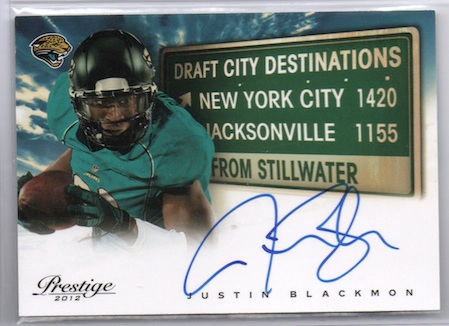This image is a horizontal, rectangular football trading card for the Jacksonville Jaguars, prominently featuring Prestige 2012 in the bottom left corner. The centerpiece is a photograph of Justin Blackman, whose name and a blue-ink signature are displayed at the bottom right of the card. Justin is depicted in the Jaguars' teal green football uniform with a black helmet, securely holding a football in his right arm while his left arm is positioned forward at a bent angle, adorned with white wrist pads and dark green gloves. His stance suggests he is in motion, looking straight ahead. 

Behind Justin is a gradient background of blue and white swirls. Over his left shoulder, to the right of the picture, is a green and white road sign reading "Draft City Destinations: New York City 1420, Jacksonville 1155 from Stillwater." The card features a silver border encompassing the entire design, with the Jacksonville Jaguar logo located on the top left. The card appears laminated, indicated by the visible plastic at the top. The image and text details are digitally or press created, enhancing the collectible nature of the card.